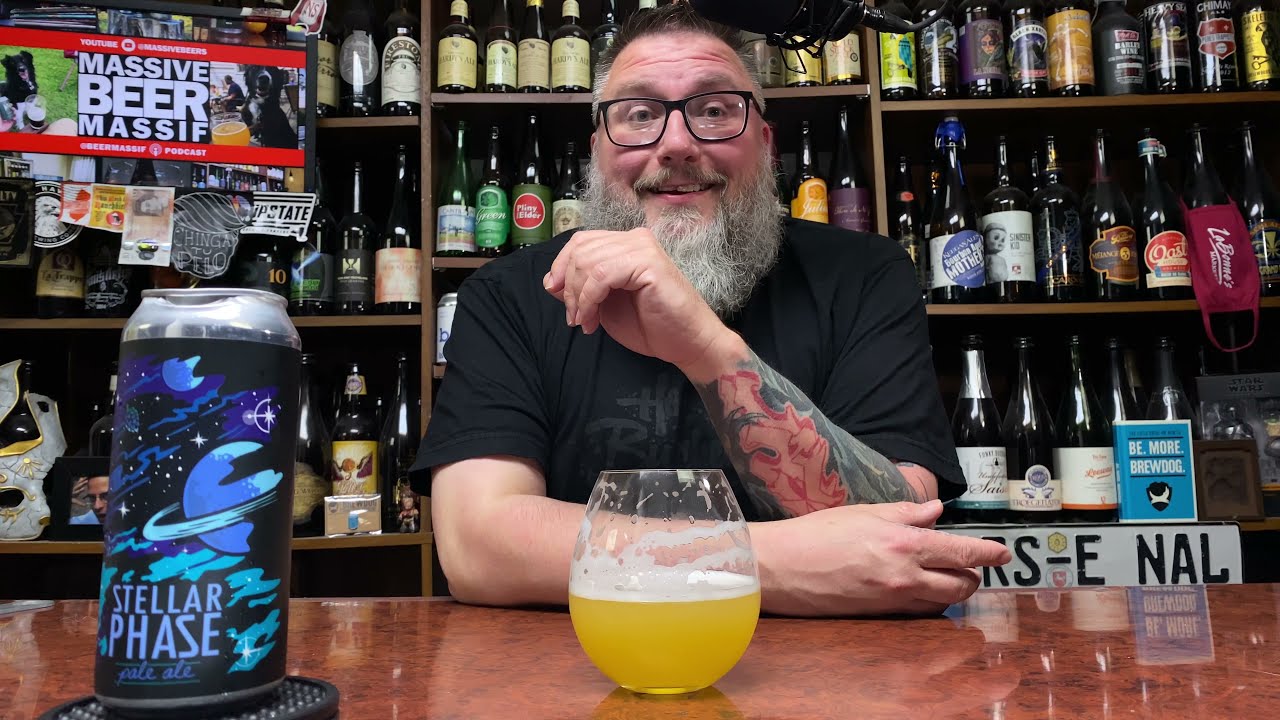This detailed image captures a middle-aged man with a salt-and-pepper beard and mustache, smiling and possibly mid-conversation, as he faces the camera. His dark hair is thinning on top and graying at the sides, and he wears black-framed glasses and a black t-shirt. He has tattoos on his left arm, which is bent with his hand near his chin, while his right arm rests on the shiny, brown marble-topped bar in front of him. A glass containing a yellow, foamy liquid, likely beer, sits on the bar directly in front of him. To the left of the glass, there is a blue can labeled "Stellar Phase Pale Ale," featuring planets and stars on its design. Behind the man, shelves filled with various beer bottles of different colors and labels span the width of the image. There are also signs visible, one to the upper left reading "Massive Beer Mastiff" and another at the bottom right of the shelves stating "Be More Brew Dog." The setting suggests a well-stocked bar or personal collection of craft beers.